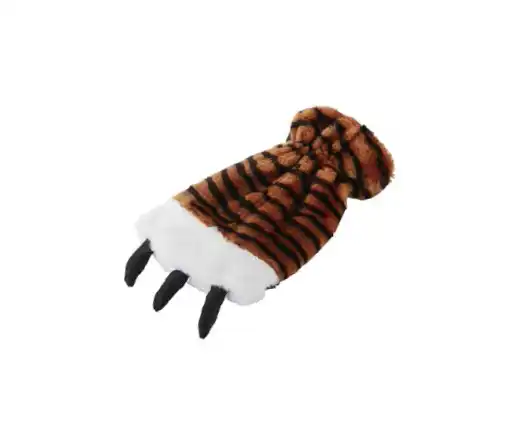The image features a warm, fuzzy glove designed to resemble a bear or tiger paw. The glove predominantly displays a brown fur pattern with black stripes, evoking a tiger's appearance. Each fingertip area is covered with soft white fur, from which three black claws extend, suggesting bear or tiger claws. The mitten includes an elastic cuff at the wrist, ensuring a snug fit without falling off. The white background accentuates the glove, making it the sole focal point in a clean, product-image style setting.